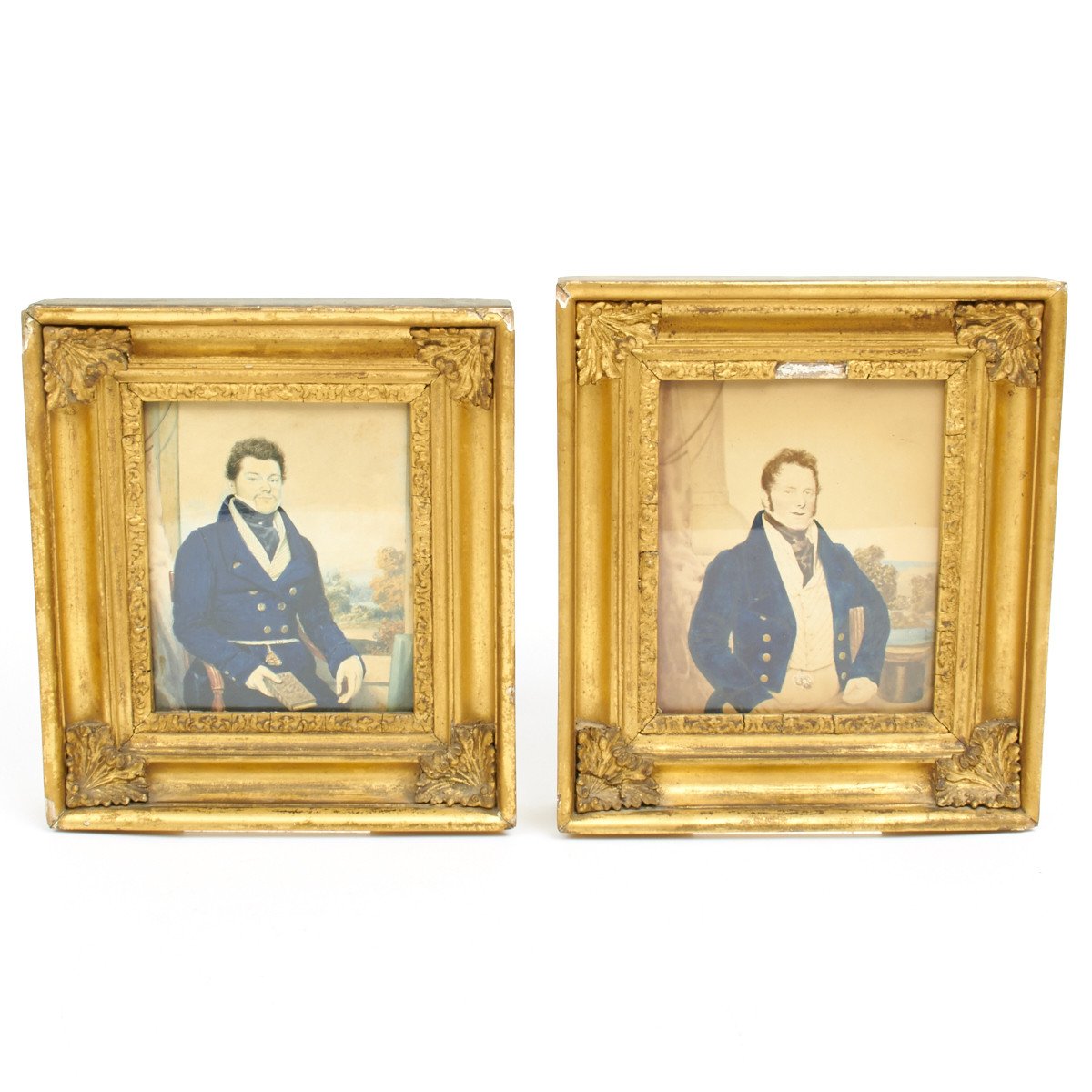This is an indoor color photograph showcasing two side-by-side framed portraits of men, likely from the late 1700s to early 1800s. Each man is depicted in a blue, double-breasted velvet coat adorned with gold buttons. They wear white pants, a white vest, and a tie around their necks. Both have brown hair with prominent sideburns. The backgrounds of the portraits are light tan, featuring various types of trees and foliage, creating a classical aesthetic. The men are seated in three-quarter view, gazing towards the camera. The portrait on the left displays a man with his blazer fully buttoned, while the man on the right has his blazer open, displaying a white shirt underneath. These framed pictures are encased in thick, ornate gold frames, with distinctive floral adornments at each corner, adding to their old-fashioned charm. The muted colors, juxtaposed with the striking blue attire, suggest that these might be tinted photographs enhancing their historical essence. Both frames show signs of wear and tear, indicating their age. The image feels like a set, possibly intended for sale on platforms like eBay.